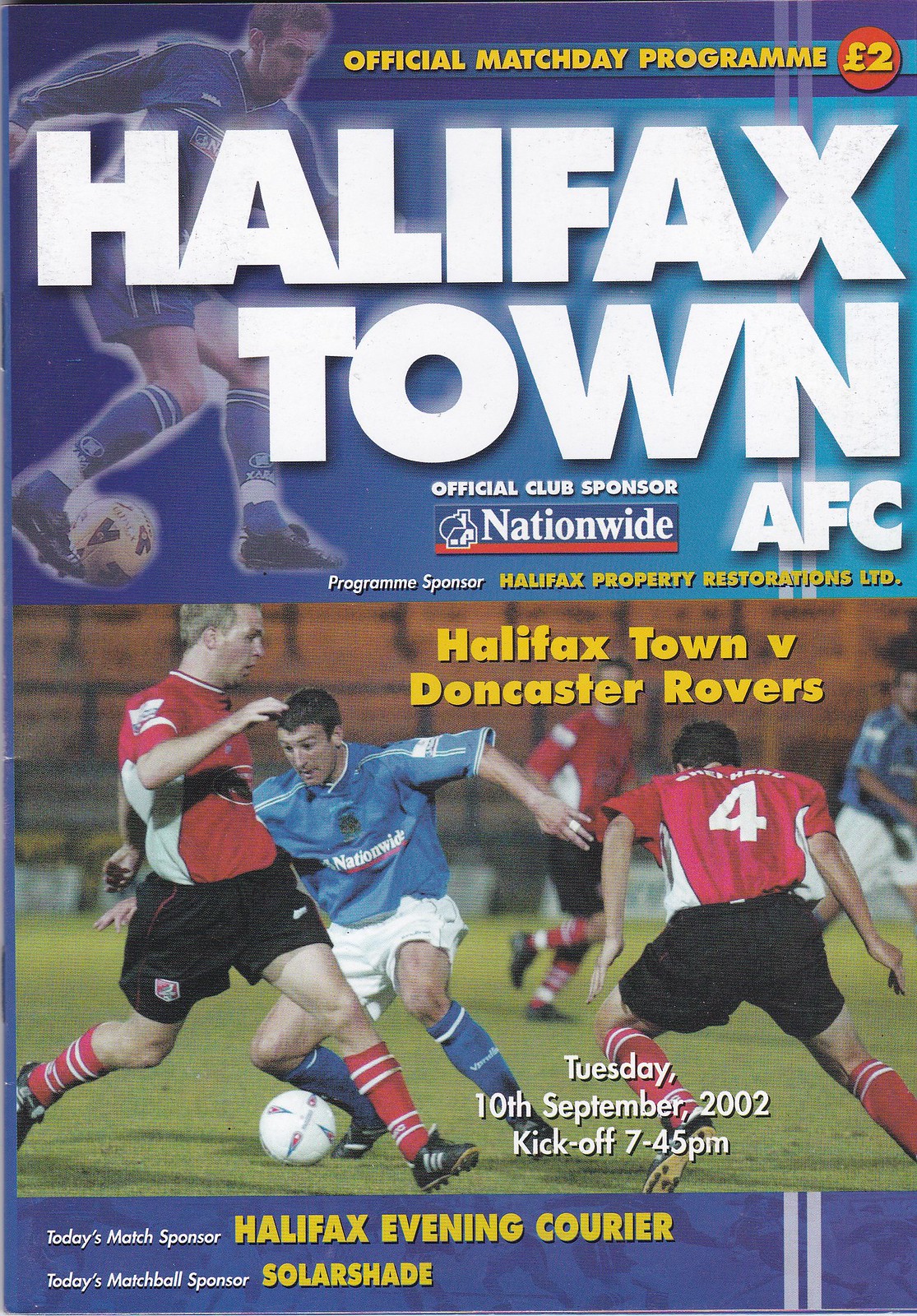The image depicts the front cover of an official match day program for a soccer game between Halifax Town and Doncaster Rovers. The program, priced at two pounds, features a prominently designed blue box at the top with yellow text reading "Official Match Day Program." A red circle within this box also indicates the cost. The main title includes "Halifax Town AFC," and acknowledges the official club sponsor, Nationwide, as well as the program sponsor, Halifax Property Restorations LTD.

Within the central portion of the cover, there is a vibrant, full-color photograph showing a moment from the soccer game. Three main players dominate the scene: two in red and white uniforms representing Doncaster Rovers, and one in a blue and white uniform emblazoned with the Nationwide logo, representing Halifax Town. The player in blue has control of the ball, which is predominantly white with green and red accents. In the background, less prominently featured, are two additional players—one in red and one in blue—positioned far from the immediate action.

At the top of the image, bold text reads "Halifax Town vs. Doncaster Rovers," while at the bottom, details about the match are provided: "Tuesday, 10th September 2002, Kickoff 7:45pm." Additional sponsors are listed at the bottom, with "Today's Match Sponsor: Halifax Evening Courier" and "Today's Match Ball Sponsor: Solar Shade."